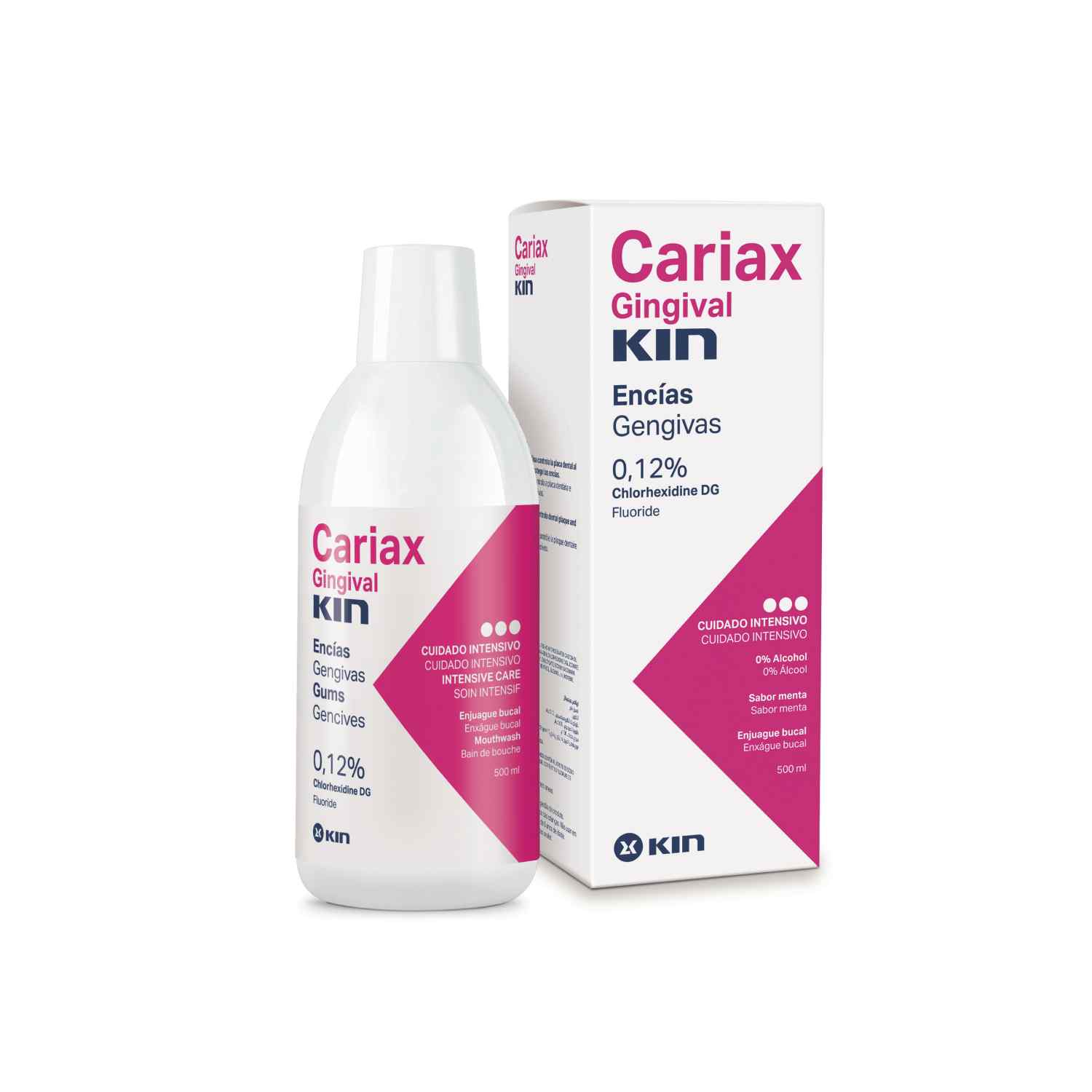The promotional photo showcases a product set against a pure white background, emphasizing its commercial intent. The product set includes a white bottle and its accompanying box, both of which feature identical minimalist design elements. Prominently displayed on both the box and bottle is a large dark pink triangle on the right side of the front. The top of the packaging is labeled "Cariax," followed by "Gingival," and "Kin" in black text. Below these titles, the product specifies its contents: "0.12% Chlorhexidine DG Fluoride," along with "Kyn Encias Gengivas" in smaller black text, indicating it might be a non-English medical or dental hygiene product. Additionally, a small circular logo with a stylized white "K" embellishes the packaging, enhancing its branding.